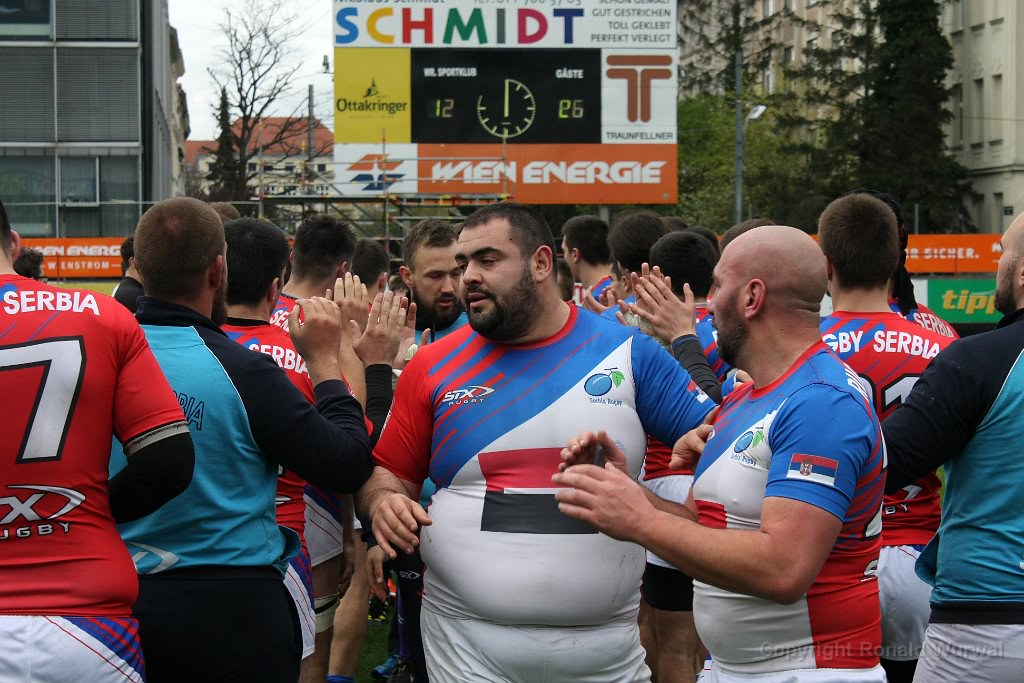The photograph captures the lively atmosphere of a sporting event, featuring participants in vibrant jerseys engaging in a celebratory moment. At the forefront, two prominent players stand out amidst the crowd, distinguished by their white jerseys adorned with accents of red and blue. One man, sporting tanned skin, short black hair, and a black beard, gazes to the left, appearing animated as he interacts with other players. On his jersey is a logo that is red at the top and black at the bottom, forming a square on the predominantly white fabric. His teammate, visible in profile, has a similar jersey, with a striking flag on the shoulder featuring red, blue, white stripes, and a crest.

The scene captures two parallel lines of participants giving each other high fives, creating a V-shaped formation. The environment is bustling, with at least a dozen people in the lines, all wearing the same colorful jerseys. Behind them, a large scoreboard is partially visible, flanked by a clock that displays the numbers '12' and '26' prominently. Above, a sign reads "Schmidt" in a mix of blue, yellow, green, and red hues. 

The background features a mix of natural and urban elements. To the right, green-leafed trees provide a touch of nature, while a leafless tree stands starkly on the center left. Buildings frame the scene on both sides: a cream-colored structure on the right and a silver building on the left. The sky overhead is overcast, casting a grayish-blue hue over the event, adding to the sense of a cool, dynamic day. The verbiage around the scene is notably in a non-English language, suggesting an international or multicultural setting.